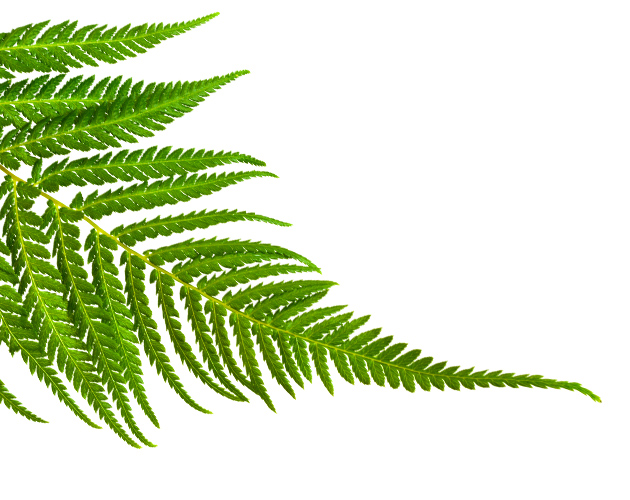The image depicts a vibrant green fern set against a pristine, all-white background. The fern frond emerges from the out-of-frame top left corner, extending diagonally down to the bottom right. The central vein or stem of the frond transitions from a lime green to a lighter yellowish shade. From this main vein, smaller leaflets sprout symmetrically on either side, mimicking the shape of the larger frond. These frondlets decrease in size as they progress toward the right, creating a tapering effect. The partially visible fern is fresh and bright, suggesting a newly sprouted, healthy plant. Adjusting from wider leaves at the top left to more narrow ones at the bottom right, the visual captures the delicately intricate structure of the fern, though the left border cuts off, preventing the full frond from being seen.